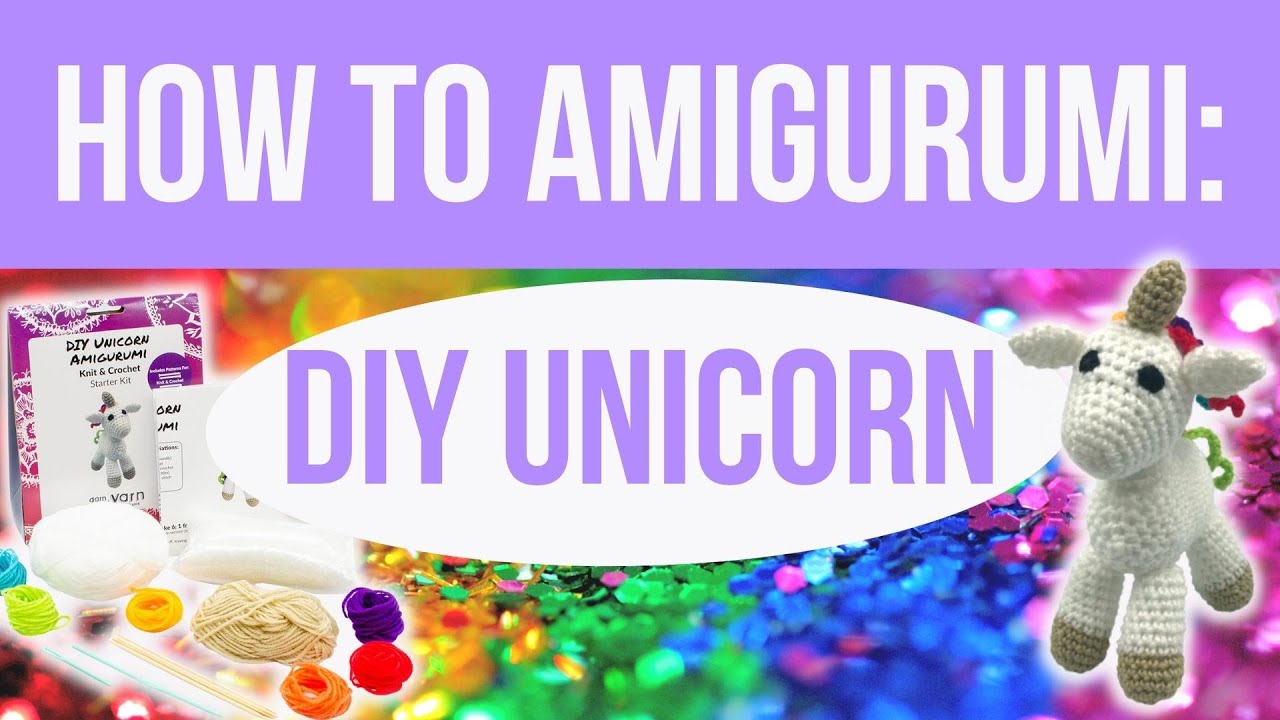This colorful graphic features a light lavender text box at the top with "HOW TO AMIGURUMI" in white, all-capital letters. Directly below this, a white oval text box with purple lettering reads "DIY Unicorn." To the right of this text box is a cute, crocheted unicorn that is predominantly white with tan hooves and a tan horn. The background is vibrant, filled with a variety of colorful yarn pieces in shades of turquoise, yellow, orange, red, and purple. There are also arts and crafts tools necessary for crocheting. Enhancing the background is a mix of rainbow-colored glitter and sparkles, adding to the whimsical feel. Additionally, to the left, there's a small book or instruction manual detailing how to create the unicorn.